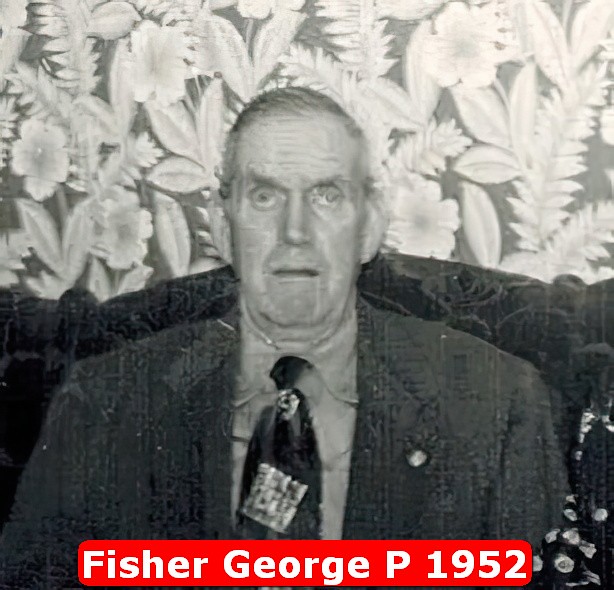The image is a grainy, black-and-white photograph of an elderly man, likely in his 70s or 80s, with a long face, dark hair, and pronounced ears. He is donned in a suit jacket, a tie, and a collared shirt, along with a small pin attached to his jacket. His facial expression appears somewhat confused or blank, with his mouth slightly open, almost as if in a grimace. His eyes are wandering off, suggesting a sense of distraction or disorientation. He is seated, possibly in a chair or couch, though the details are unclear due to the image's poor quality. Behind him, the wall is adorned with floral wallpaper featuring stark white, gray, and black flowers and leaves. At the bottom of the photograph, a red banner with white text reads "Fisher George P. 1952." The overall image evokes a sense of old-fashioned, professional portraiture but is marked by its graininess and worn condition.